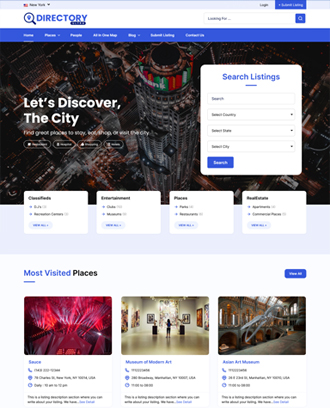This image features a predominantly white background with a structured layout. At the top, there is a gray header that includes a search bar, which is composed of a blue square with a white magnifying glass icon. Below the header, there is a large, vibrant image of a cityscape at night, showcasing numerous tall buildings illuminated by lights. Overlaid on the city image is the text "Let's Discover the City" in white.

Beneath the cityscape image, there is a white box containing the phrase "Search Listings" in blue text. Further down, the layout includes a series of rectangular sections aligned vertically. The first of these sections contains a prominent blue rectangle with the word "Search" in white. Below this, there are four white squares labeled "Most Visited Places" in blue and black text. 

The section also includes three smaller images. The first image has a blue caption underneath it labeled "Seen." The second image is titled "Museum of Contemporary Art," again in blue text. The final image appears to be of an Asian art museum, though the exact name is unclear. The overall design effectively directs the viewer's attention to explore city listings and highlighted attractions.